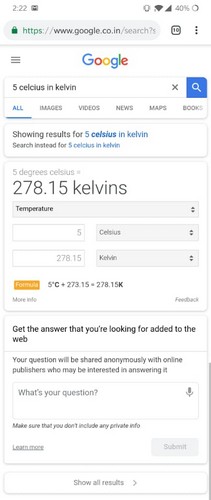A screenshot captured from a Google search shows the query "5 Celsius in Kelvin" entered in the search bar. At the top of the image, the Google URL is clearly visible. The search results include a prominently displayed calculator which dynamically converts temperatures. The calculator shows the conversion result, stating "5 degrees Celsius equals 278.15 Kelvin." Below this line, there is a drop-down menu labeled "Temperature," allowing users to select different units for conversion. On the left side of the calculator, the input value "5" is linked to another drop-down menu on the right, which is set to "Celsius." Directly below, another set of values appears: "278.15" on the left, linked to a drop-down menu on the right side set to "Kelvin."